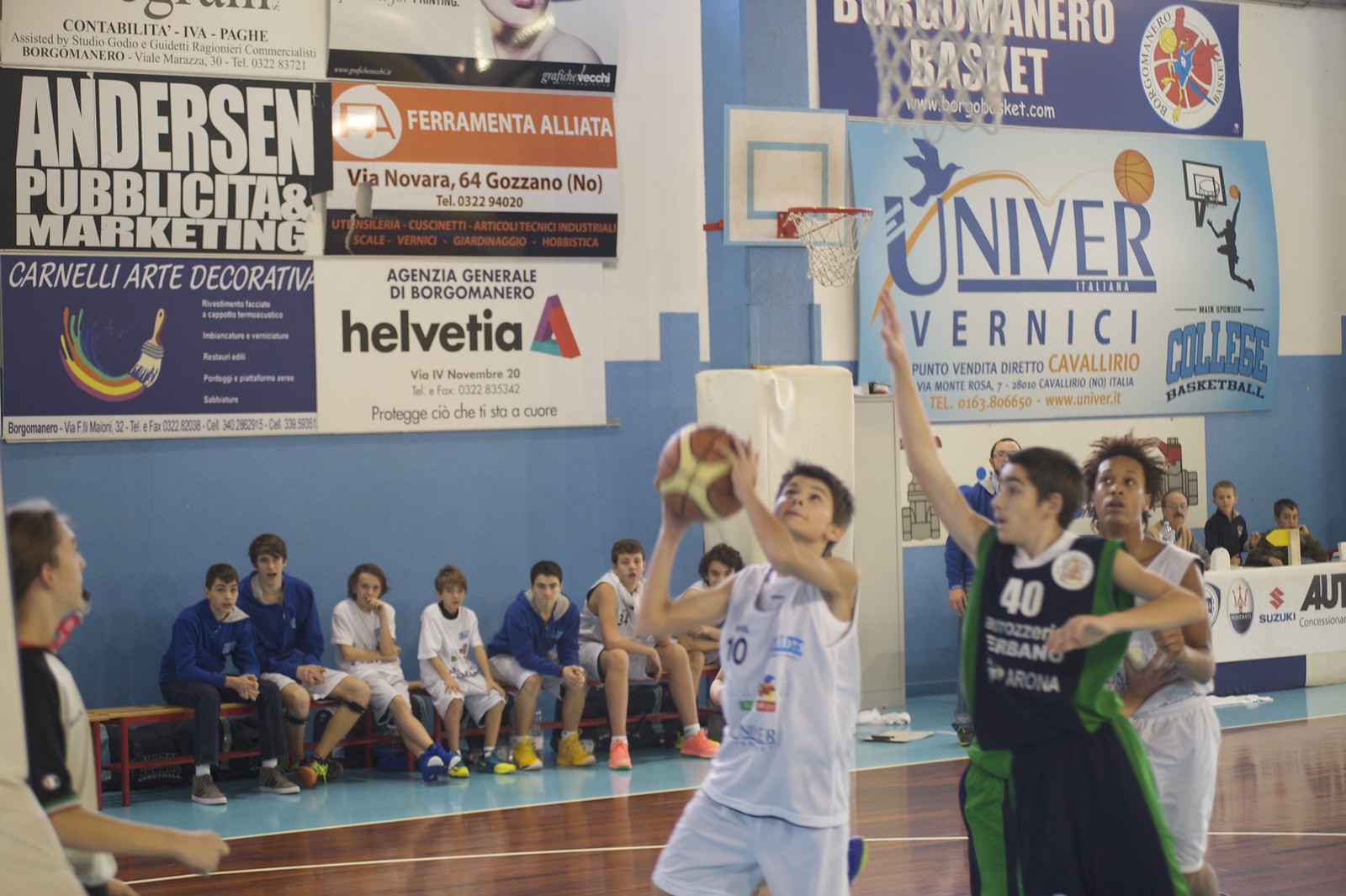The photograph depicts an intense children's basketball game in a gymnasium with blue walls and a dark wood court. In the foreground, a young boy in a white jersey and white shorts, possibly around 12 or 13 years old, is poised to take a shot, holding an orange and cream-colored basketball. Next to him, an opposing player in a dark blue jersey with green trim and the number 40 in white, is attempting to block the shot with his left hand raised and his right hand outstretched for balance. Another teammate of the boy in white, dressed similarly in a white jersey and shorts, watches the action unfold.

To the bottom right corner of the image, a referee, with black hair and wearing a gray shirt with black shoulder trim, holds a whistle in their mouth, appearing ready to make a call. Above the court, a series of advertisements adorn the blue wall. There's a large sign composed of four smaller sections: a black sign with white text, an orange and white sign, a white sign with the text "Helvetia" in black, and a dark blue sign featuring a paintbrush logo with multiple colors and white text. Another large sign reads "Univer" in dark blue, accompanied by a silhouette of a man jumping to dunk a basketball, placed above a dove symbol.

In the background, a group of about seven students sits on a bench, closely following the game. Above them, you can see an old basketball hoop with a white and blue backboard and a red rim, adding to the dynamic atmosphere of the gym. Additionally, a table draped in a white tablecloth with a mix of adults and students is visible, underscoring the community's engagement in the game.